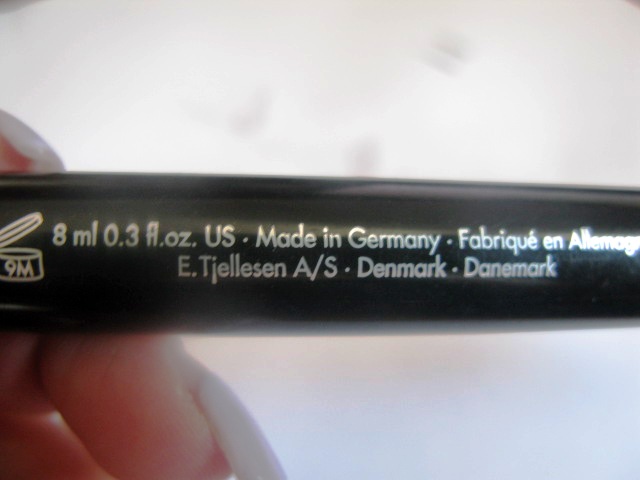In this detailed color photograph, a woman’s hand adorned with long white fingernails is seen holding a makeup product at the left edge of the image. The elegant manicure is prominently displayed as the hand delicately grasps the item, which is primarily out of the frame, revealing only limited text. The visible text on the makeup item indicates it is black in color and highlights crucial details such as '8 ml' (0.3 fluid ounces), manufactured in Germany, and additional information in French noting 'fabriqué en Allemagne' as well as mentions of Denmark 'Danemark'. A small, open jar icon is located at the far left of the frame, clearly marked with '9M,' signifying that the product remains usable for nine months once opened. The entire scene is set against a pristine white background, emphasizing the simplicity and elegance of the captured moment.